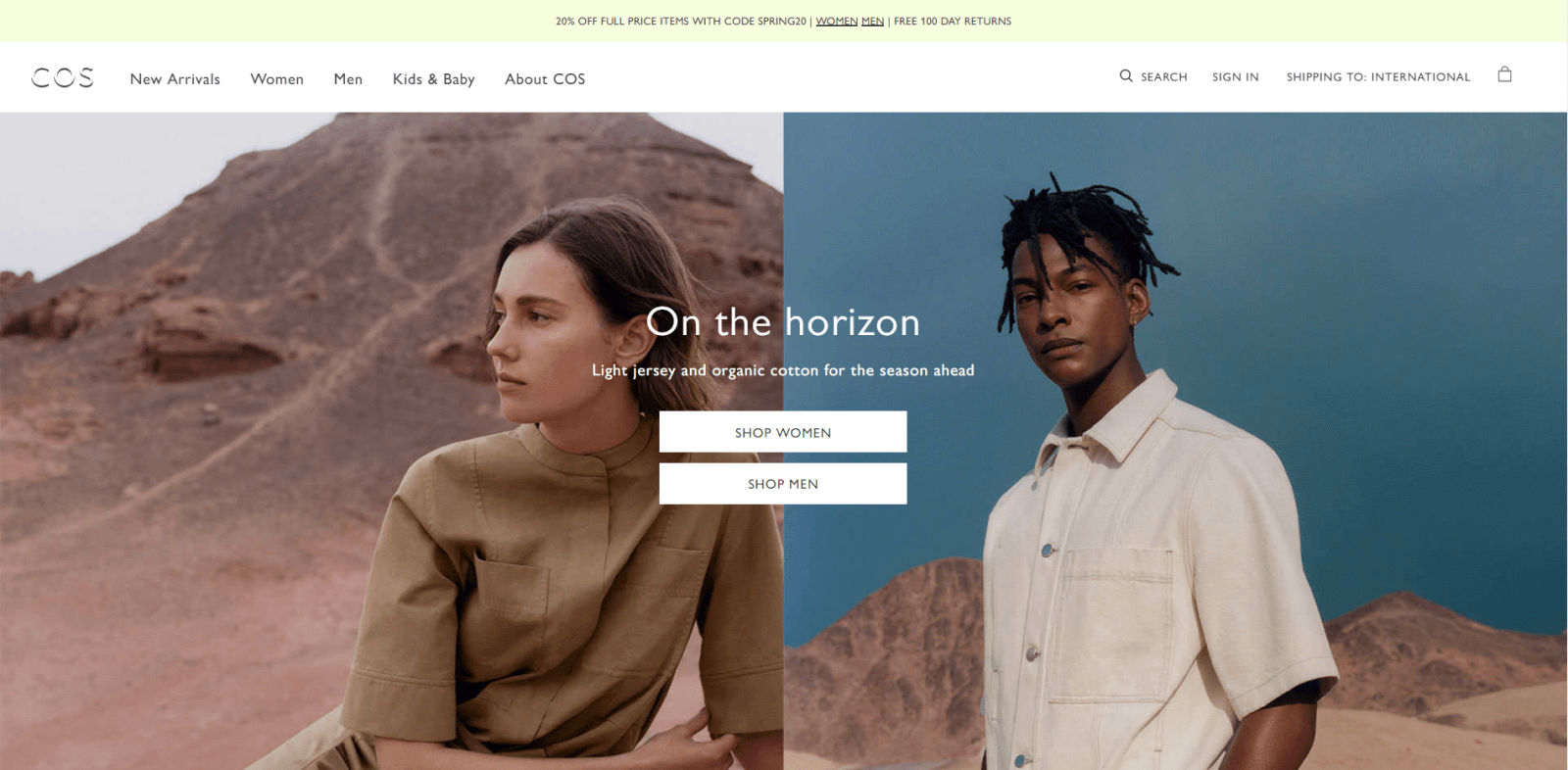The webpage features a minimalist, mint-green banner at the top, extending across the entire width of the screen. Centered within this banner is bold, black text announcing "30% off full price items with code SAVINGS," followed by a dividing line. Adjacent to this line is additional black text comprising two sets of words, the second set having four words, although they are too blurry to decipher.

Below this banner is a navigation bar set against a white background. From left to right, it includes the following clickable options: "COS," "New Arrivals," "Women," "Men," "Kids & Babies," and "About COS." A marginal space leads to the right-hand side where search and user account icons reside. Here, "Search," "Sign In," and "Shipping to International" are written, accompanied by a small shopping bag logo.

The main body of the webpage highlights two side-by-side images. The left image features a Caucasian girl with shoulder-length brown hair, dressed in a brown mandarin-collared shirt with dual pockets on the chest. She gazes to the left, standing against a backdrop of brown rock and open sky. The right image showcases an African American man with short, ear-length dreadlocks or braids. He is attired in a white button-up shirt with a left breast pocket, similarly posed in front of brown rock formations with the sky behind him.

Centered between the two images, bold text announces "On the Horizon." Below this, subtler text describes the collection: "All written by Light Jersey and Organic Cotton for the season ahead." Two horizontally aligned white bars beneath these texts prompt users to "Shop Women" and "Shop Men" respectively.